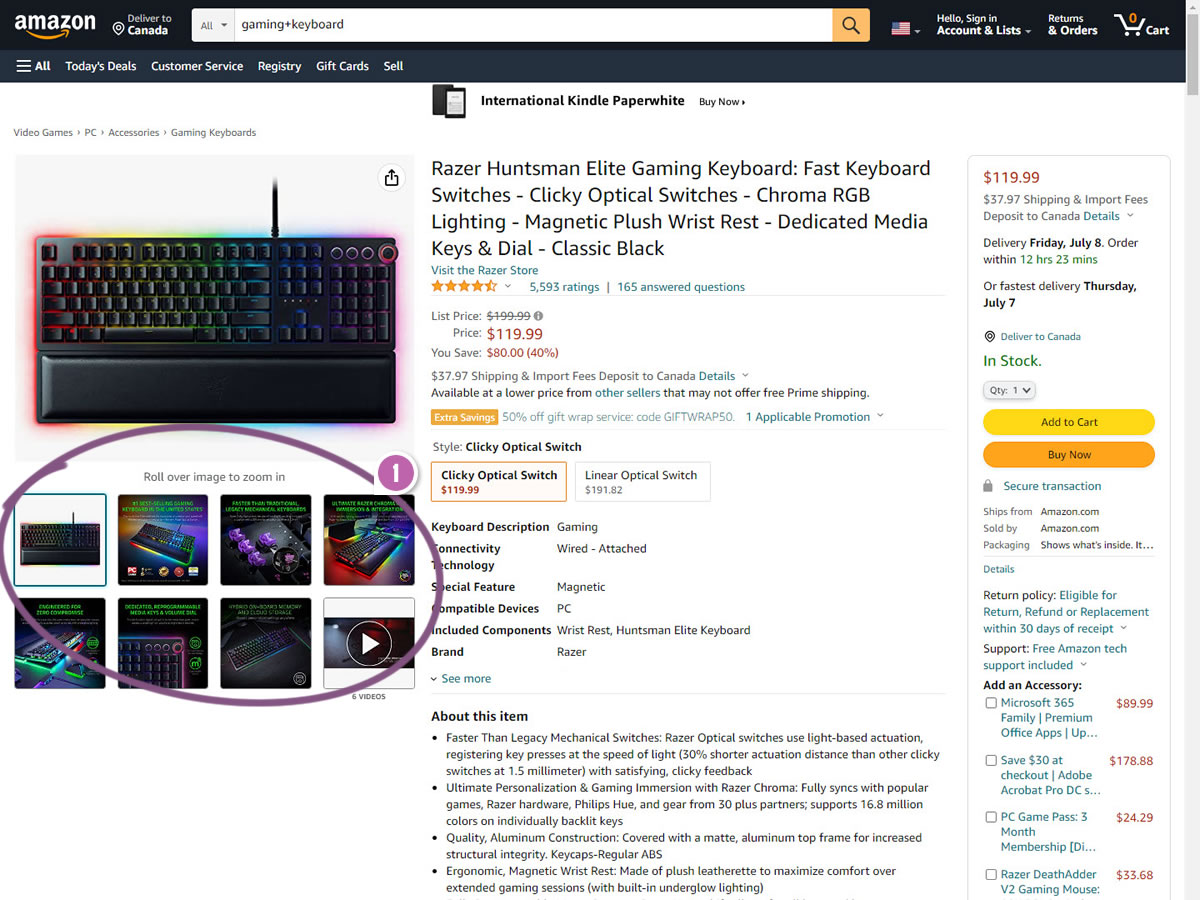On an Amazon pitch page for a gaming keyboard, the user is searching for "laptop keyboard". At the very top of the page is a long black navigation bar featuring the Amazon logo on the upper left and the text "Deliver to Canada" in white letters to the right. In the center of this bar, there's a large white search box with a gray square and the word "All" in black letters alongside a downward-facing triangle. Towards the left of the search bar, you see the search terms "gaming and keyboard" in the box. To the right of this are several icons and text, including an orange box with a black magnifying glass, a faint American flag, and "Hello, Sign In, Account & Lists" in white letters. Next to these are "Returns & Orders" and a shopping cart icon displaying an orange "0" and the word "Cart". Below this black bar runs a dark gray bar with clickable options labeled in white: "All", "Today's Deals", "Customer Service", "Registry", "Gift Cards", and "Sell".

The image on the page showcases a gaming keyboard, specifically the Razer Huntsman Elite. In the upper left, there is a square image of the keyboard set against a gray background. The keyboard is black with under-lighting featuring shades of orange, yellow, blue, and purple. Below this image are several smaller rectangular images of keyboards, encircled by a purple hand-drawn box with a white number "1". Above these smaller images is the instruction, "Roll over image to zoom in".

Central to the page is a detailed product description. At the top, in large black letters, the text reads: "Razer Huntsman Elite Gaming Keyboard, Fast Keyboard Switches, Clicky Optical Switches, Chroma RGB". Subsequent details include "Lighting - Magnetic Plush Wrist Rest, Dedicated Media Keys and Dial, Classic Black", followed by extensive product information and specifications.

To the right of the product description, a tall white bordered box displays the price: "$119.99" in red letters. Below the price, in gray letters, it mentions a $37.97 shipping fee and import fees to Canada, with further details available in blue letters. The availability status and fastest delivery options are listed, alongside buttons for adding to the cart (yellow with black letters) and buying now (orange oval with black letters). Below these buttons are options for a secure transaction, the return policy, and additional accessories with associated costs, such as Microsoft 365 family, indicated by red numbers next to checkboxes.

This detailed page suggests a Canadian video gamer or enthusiast searching for a high-quality gaming keyboard to purchase from Amazon.